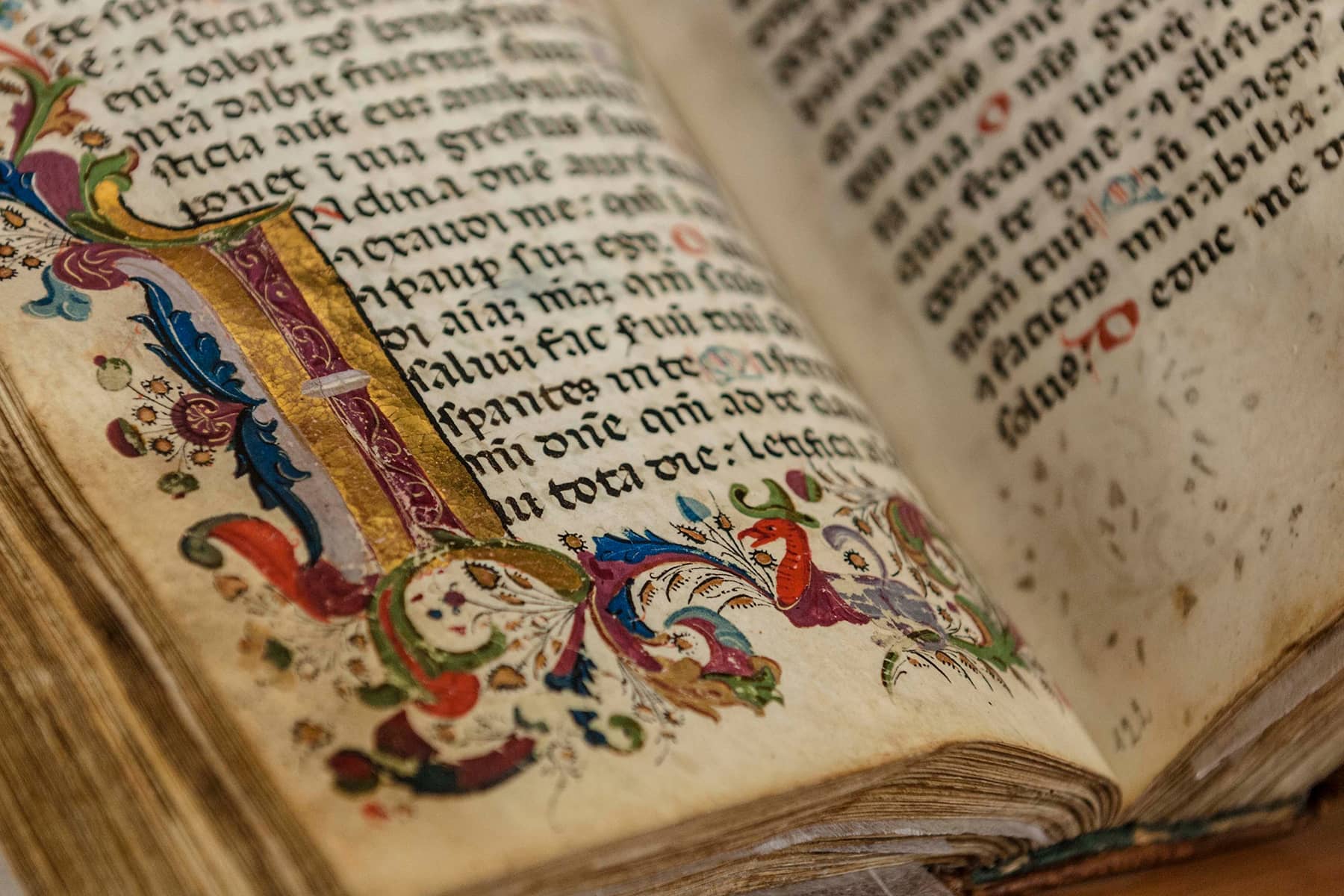The image showcases a close-up of an old, possibly medieval book, with pages yellowed and browned with age. The text, written in bold black letters, is in an unknown non-English language, possibly Latin. The ornate decorations on the left side of the page are rich in detail and color, featuring medieval patterns with intricate curvy designs, including vines, leaves in greens, gold, blues, and reds, and whimsical elements such as a red dragon wearing a green wizard hat. Prominently, there is a large, golden 'H' adorned with elaborate artistry, enhancing the historical and artistic value of the image. The photograph focuses on this elaborate edge, highlighting the florals, gold accents, and the overall antique quality of the book.